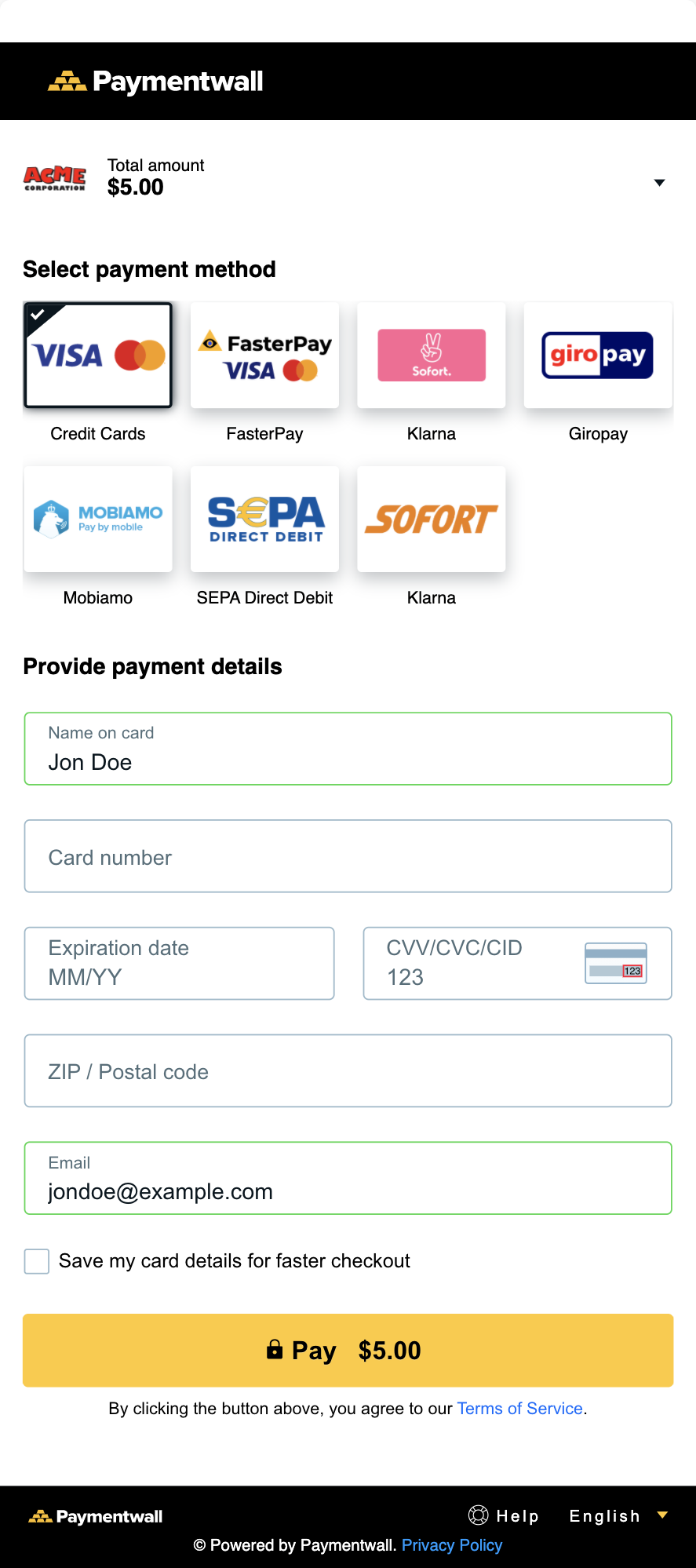**Image Description: Acme Landing Page**

The image depicts a landing page for Acme's online payment portal. On the left side, there is a prominent "Acme" logo in bold red letters, with an unreadable word beneath it. The total amount of the transaction is displayed as $5. 

At the top of the page, a black banner spans the width, featuring a white "Paymentwall" logo with a brown triangle icon adjacent to it. 

Under this banner, the text "Select Payment Method" is displayed, followed by several payment options including Visa, FasterPay Visa, Giropay, Sofort, SEPA Direct Debit, Moblamo, and Klarna.

Below this section is a form titled "Provide Payment Details" in black text. The form includes fields for various pieces of information:
- "Name on the Card": Pre-filled with "John Doe"
- "Card Number": Blank 
- "Expiration Date": Blank 
- "CVC Number": Pre-filled with "123"
- "Zip Code": Blank 
- "Email": Pre-filled with "johndoe@example.com"

A checkbox option is provided to "Save my card details for a faster checkout."

At the bottom of the form, an orange banner with a lock padlock secure icon displays "Pay $5." Beneath this button is a disclaimer that reads: "By clicking the button above, you agree to our terms of service."

Finally, the page concludes with a black footer displaying "Paymentwall" and "Powered by Paymentwall," along with links for Help, Privacy Policy, and a note indicating the language as English.